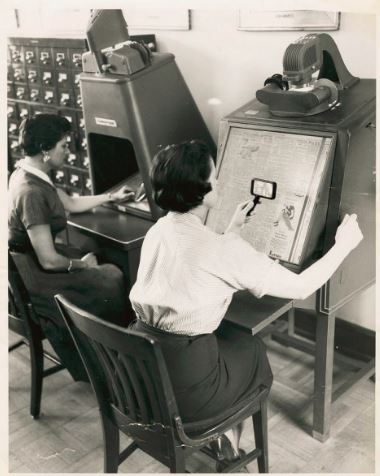A vintage black and white photograph captures two women sitting in a library, each positioned at large microfilm machines. The woman closest to the camera, identifiable by her white short-sleeved blouse tucked into a dark skirt, is seated on a wooden chair. She holds a rectangular black magnifying glass in her left hand, focusing it on the microfilm displayed in front of her, while her right hand operates a crank on the machine. To her left, another woman, dressed in a dark-colored dress with a white collar, peers into her own microfilm machine. Both women are intensely engaged in their work, highlighting the meticulous nature of archival research during that era. The machines themselves feature a square metallic frame with a triangular door that opens up, further emphasizing their vintage design and function.